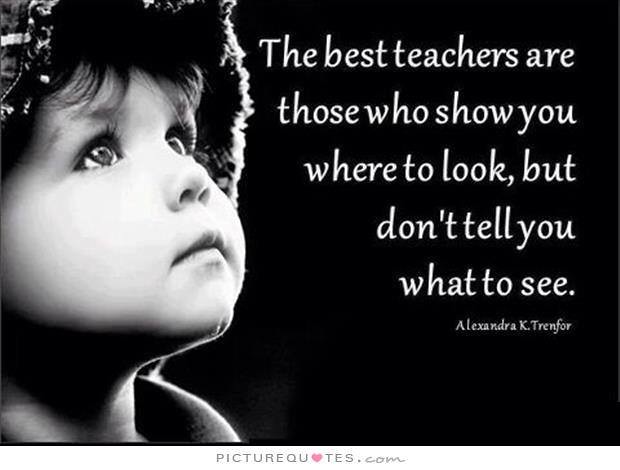This horizontally aligned black and white poster features a close-up image of a young child, likely Caucasian, looking plaintively upwards, with visible long eyelashes, beautiful eyes, a cute pudgy nose, and soft lips. The child is wearing a winter hat, with a few wisps of blondish or brownish hair peeking out on their forehead. Positioned on the left side, the child's eyes are fixed intently towards the right. On the right side of the poster, white text is right aligned over five lines, stating, "The best teachers are those who show you where to look but don't tell you what to see." Below the quote, the name "Alexandra K. Trenfor" is attributed. The background on this side is a solid black, creating a striking contrast with the text. Additionally, beneath the image, there is a white trim area featuring the text "picturequotes.com," with the 'O' in quotes replaced by a red heart.